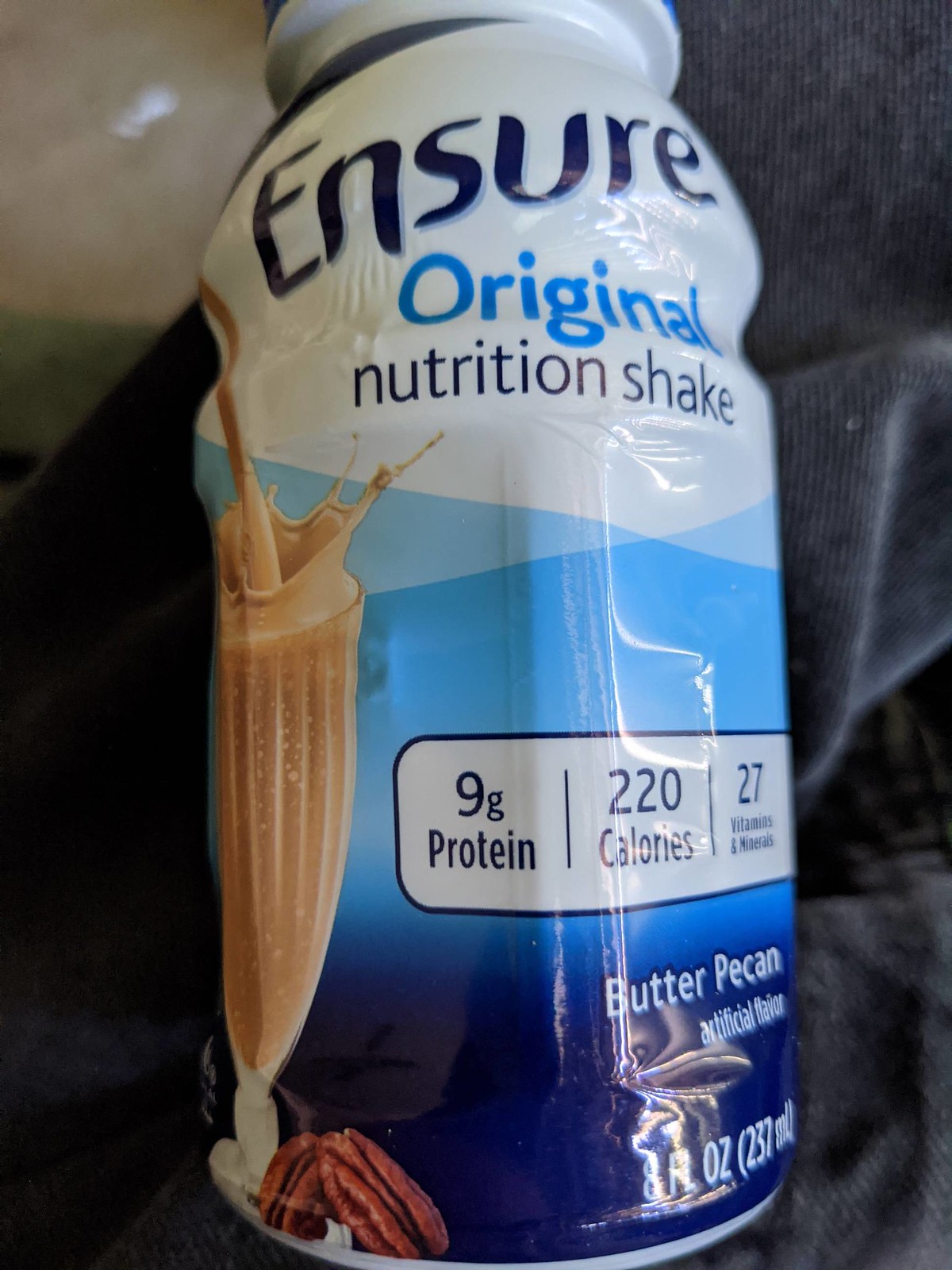The image features a close-up, color photograph of a plastic bottle of Ensure Original Nutrition Shake in a portrait format. The bottle, primarily white and blue with shades ranging from light to dark, carries a label that prominently displays the text: "Ensure Original Nutrition Shake" along with nutritional information: "9 grams of protein, 220 calories, and 27 vitamins and minerals." The flavor is specified as butter pecan, noted to be artificial. The front of the label also showcases a tall, clear glass of milkshake being poured, with liquid splashing into it, accompanied by images of pecans in the lower left corner. The bottle is 8 fluid ounces (237 milliliters) in size. The background hints at a setting where the object is placed on a gray cloth or possibly resting in someone's lap, with a glimpse of black jeans or a black jacket visible.